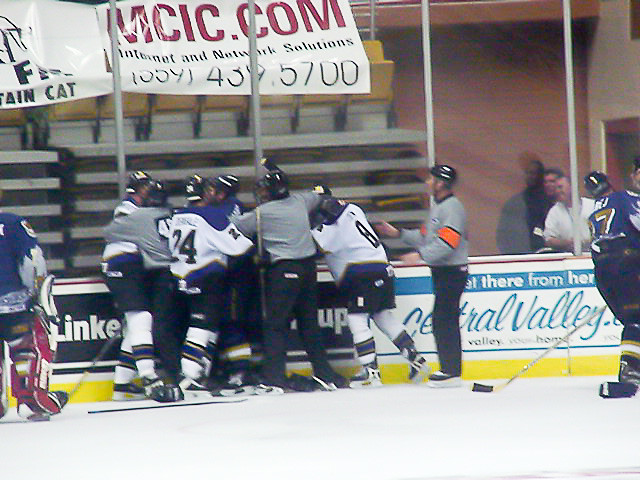In this image taken at a hockey game, a scuffle involving several players unfolds near the sideboards in the left midsection of the rink. The players are distinguishable by their jerseys: some are white with blue accents and blue numbers, including numbers 24 and 8, while others wear blue jerseys with red gear and gold numbers. Three referees are actively involved in managing the altercation; two are grabbing players while one stands outside the fray. The referees are dressed in gray shirts with orange armbands and helmets. Additional players and coaches are seen converging from both sides, and one hockey stick lies abandoned on the ice.

The spectators' section in the background features grey seats with yellow tops, currently empty but with some seats folded up. Through the glass panes, three men observing the scene can be seen. Signage around the rink includes advertisements for centralvalley.com and LinkedIn. A red and white banner also hangs in the background.